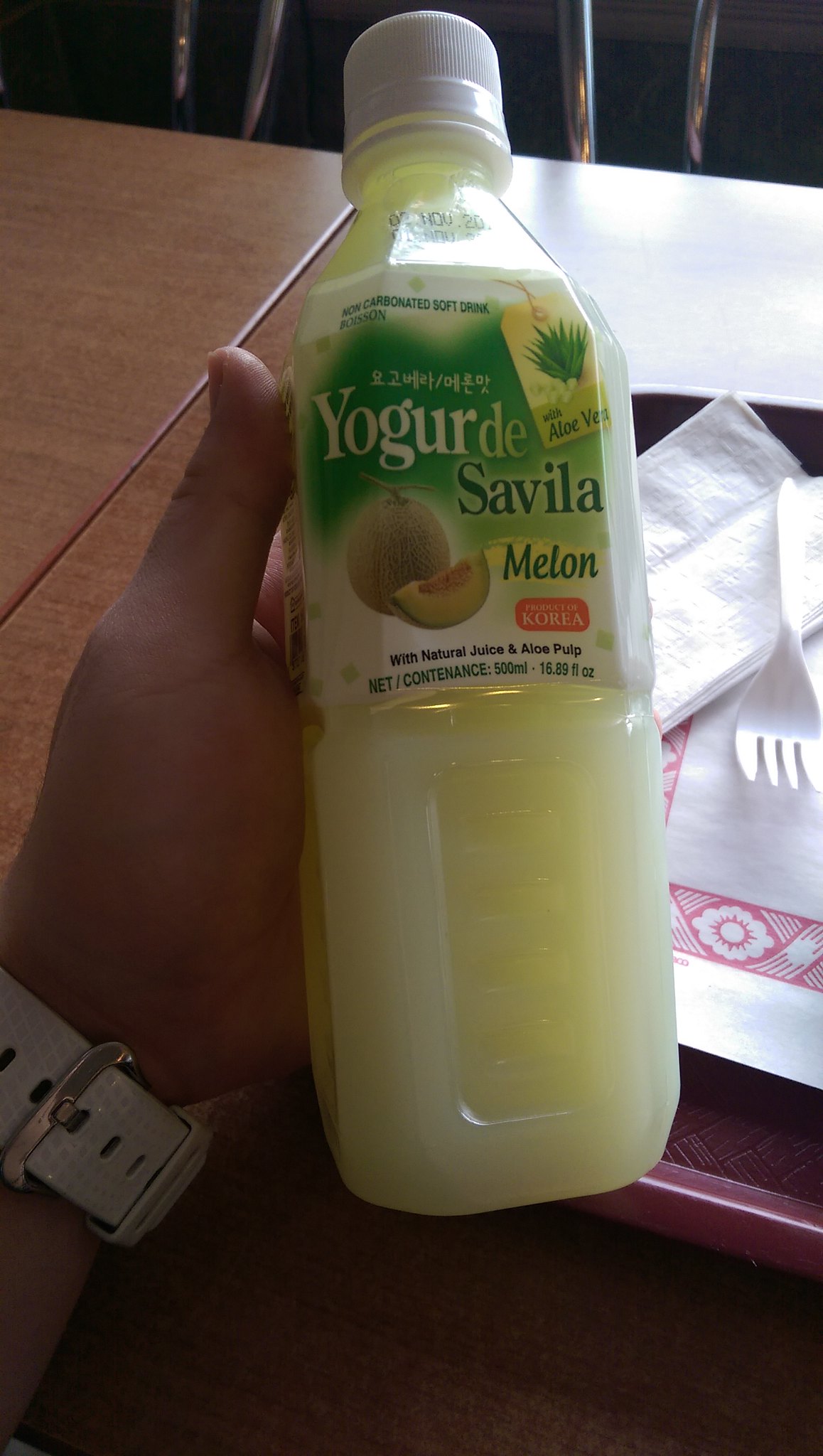The photo depicts a left hand, likely feminine and of Caucasian complexion, adorned with a white leather wristwatch, holding a sealed plastic bottle with a white cap. The bottle, labeled "Yogurt de Sevilla," contains a milky white liquid and features a green and white label highlighting flavors of melon and aloe vera. The label depicts a cantaloupe image and includes Korean writing, indicating it is a product of Korea, with additional text mentioning natural juice and pulp. In the background, the bottle rests on a maroon food tray placed on a dark wooden table, accompanied by a white plastic fork, a white napkin, and a tray liner with red detailing. The setting resembles a lunchroom, with glimpses of chair legs at the top of the image and sunlight filtering into the frame, which appears slightly blurred and narrow, as if taken with a cell phone.